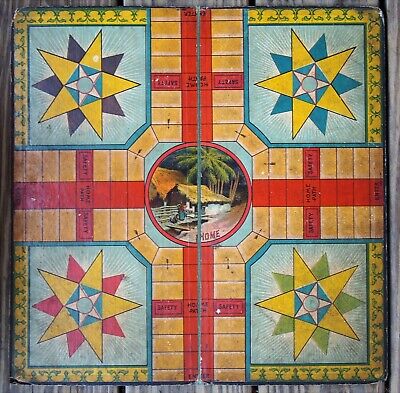The image depicts a detailed, square-shaped wooden board, reminiscent of a game board, similar to Ludo. The board features star-shaped designs at each of its four corners, each star distinguished by different colors: tan, red, green, yellow, blue, and dark blue. A prominent red cross intersects the board, running horizontally and vertically, connecting the stars and breaking the board into sections. The main body of the board is divided into rectangular columns, some in red and others in light brown. 

At the very center of the board is a detailed illustration of a beach scene, featuring a small shack or hut with accompanying palm trees and a boat situated on the shore. Below this illustration, the word "HOME" is inscribed. The entire board is laid out on a visible grey-colored wooden surface. The intricate details and colorful elements of the board create a visually engaging and intricate design.